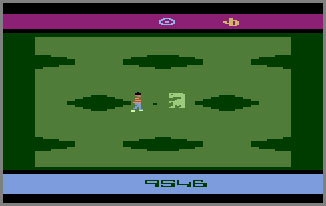This image is a screenshot from the notorious E.T. the Extra-Terrestrial video game for the Atari 2600, widely regarded as one of the worst games of all time. The screenshot exhibits a simplistic, 8-bit design typical of its era. At the top of the image, there's a purple strip featuring a blue circle with a blue dot inside it and an adjacent yellow or orange symbol. The bottom of the image displays a score of 9546 in dark green against a blue background strip. The central part of the image showcases a lighter green field on a darker green backdrop. Positioned in the center is a small, pixelated character with black hair, fluorescent green shoes, blue jeans, and a red and white striped top. This character is facing a light green, E.T.-like creature, reinforcing the game's connection to the famous 1982 movie.